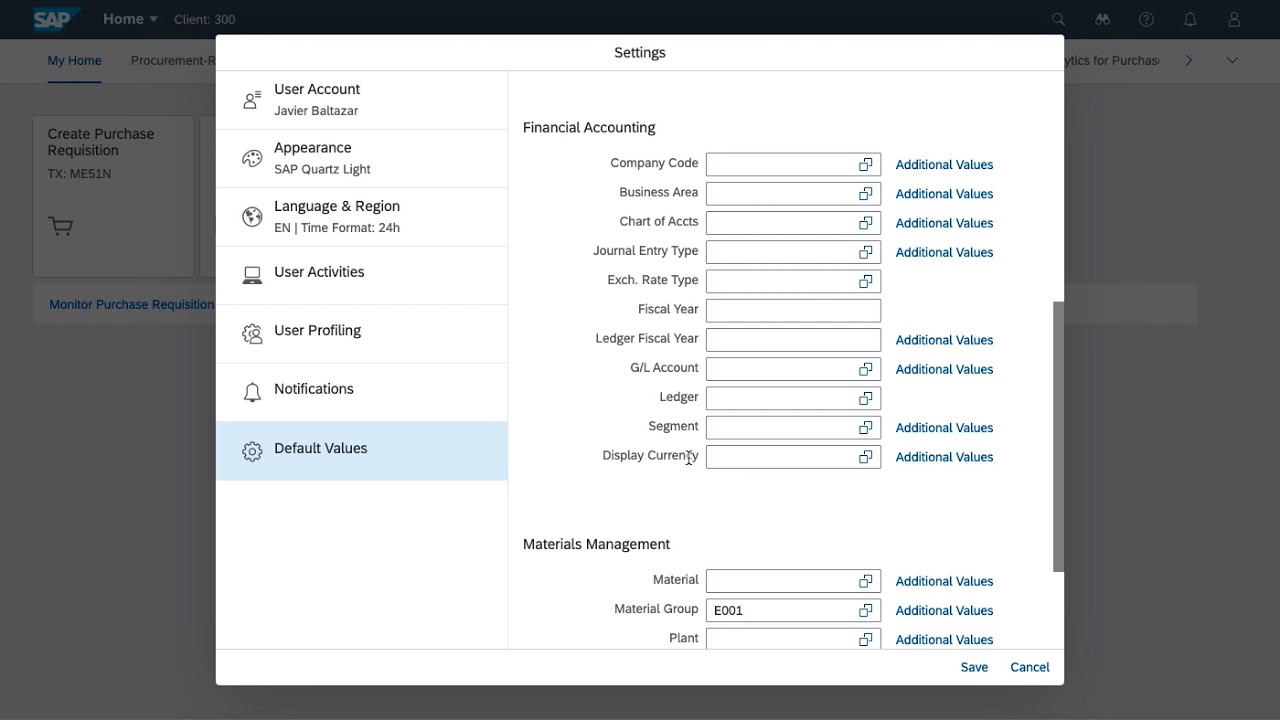**Caption:**

The image is a screenshot of a web interface under the category "Websites." At the top, there is a black border line. On the top left corner of this border, the "SAP" logo appears in white letters with a blue trim. Next to the logo, the word "Home" is visible, accompanied by a down arrow which suggests additional options can be accessed. Directly below this, the navigation bar displays "My Home" and "Procurement." Further down, there are options for "Create Purchase Requisition" and "Taxes," the latter represented by a cart icon. "Monitor Purchase Requisition" is also listed.

A pop-up window partially obscures the lower part of the page, restricting visibility of other content. The pop-up’s left-hand side includes several user settings: "User Account: Javier Baltazar," "Appearance: SAP Quartz Light," "Language and Region: EN," "Time Format: 24 Hours," "User Activities," "User Profiling," and "Notification." Currently, the "Default Values" option is highlighted in the pop-up.